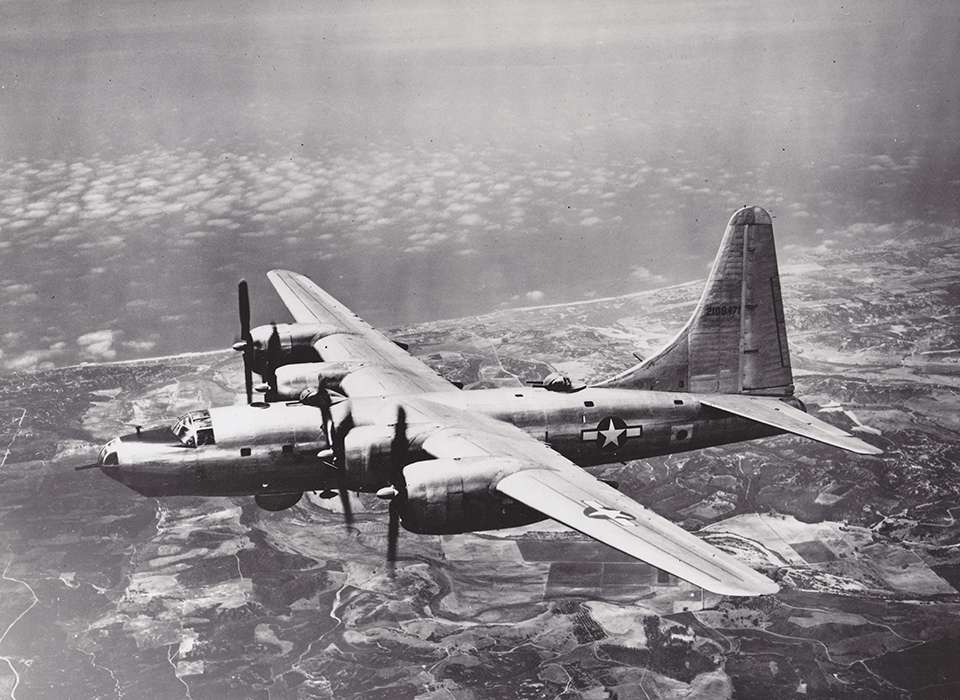This black-and-white photograph, likely from the 1930s or 1940s, captures a World War II-era military aircraft soaring high above a varied terrain of fields and open spaces. The airplane, a large four-engine bomber with propellers, prominently features a U.S. Air Force star insignia on its side and wing. It has a distinctive tail fin and wings positioned above its fuselage. Visible are its front landing wheels, nose-mounted gun, and an additional turret near the back of the plane. The scene is set against a backdrop of scattered clouds, with far-reaching views of the landscape below, suggesting a mix of barren land, farmland, and possibly some faint outlines of roads and buildings.